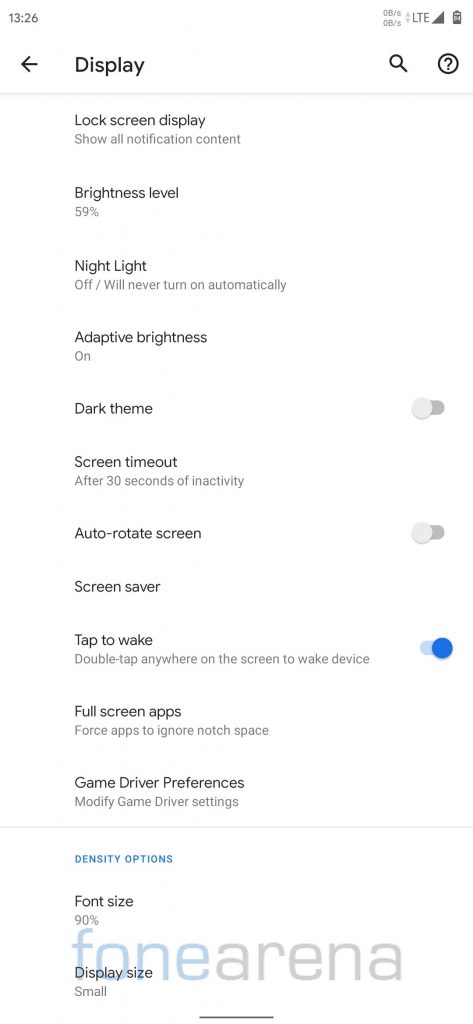A screenshot taken on an Android phone, showcasing its display settings menu. At the bottom right corner, there is a watermark from "Fone Arena." The settings displayed include:

- **Brightness Level:** Set to 59%
- **Night Light:** Off
- **Adaptive Brightness:** On
- **Dark Theme:** Off (with a toggle to turn it on)
- **Screen Timeout:** Set to 30 seconds of inactivity
- **Auto-Rotate:** Off
- **Screen Saver:** Option available for further customization
- **Tap to Wake:** On
- **Full-Screen Apps:** Requires a click to access additional settings
- **Game Driver Preferences:** Allows modification of GPU settings on the chipset
- **Font Size:** Set at 90%
- **Display Size:** Small

The interface features a white background and black text, consistent with the dark theme being turned off. The auto-rotate function is disabled, meaning the screen orientation will remain static unless adjusted within an application.